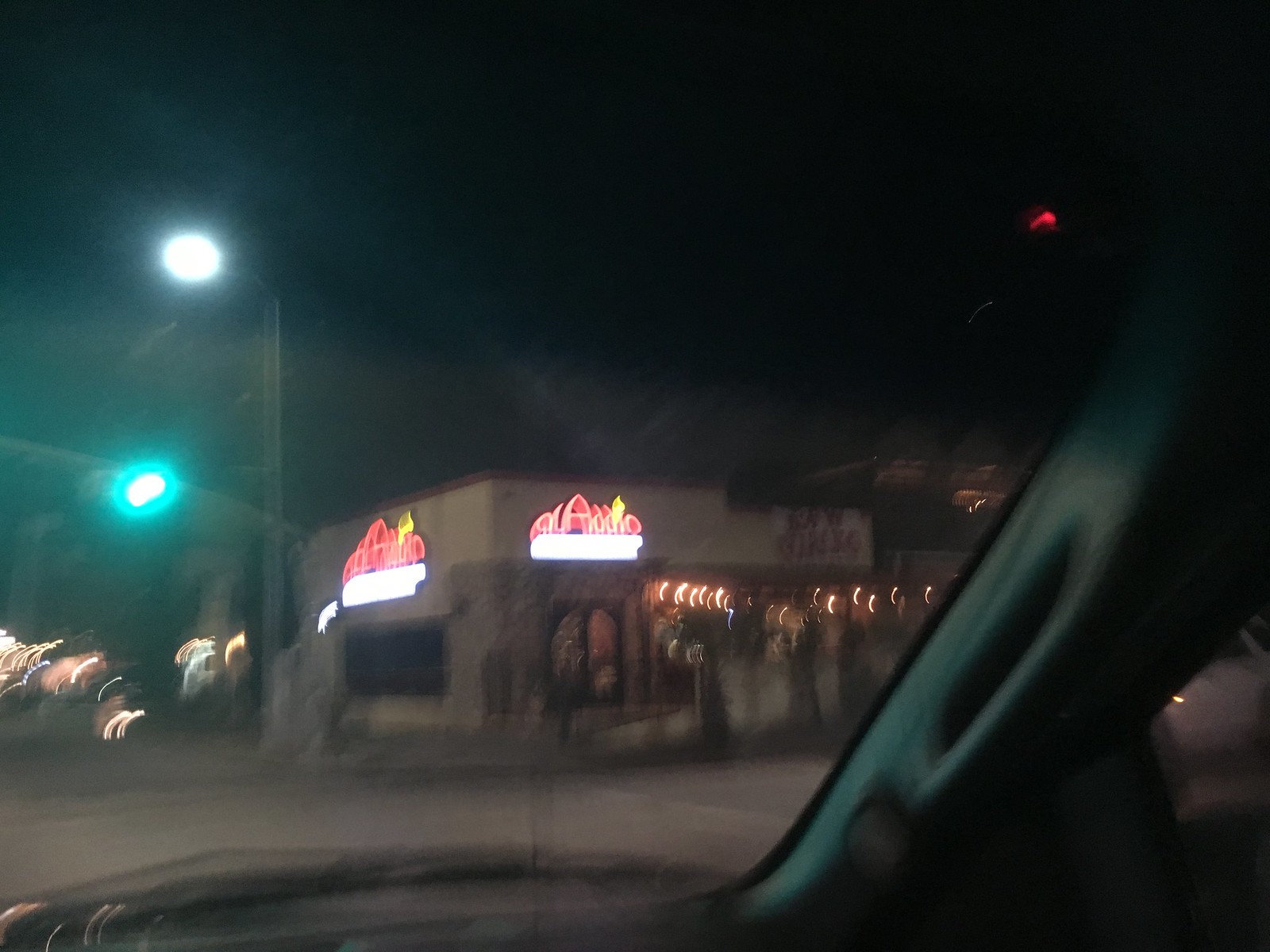This nighttime photograph, captured from the passenger seat of a vehicle, provides a blurry yet atmospheric view of a street corner. Through the windshield and over the black car hood, illuminated by streetlights and street reflections, a restaurant stands as the focal point. The brown, possibly adobe-style building features neon signage with red and yellow letters on the front and left side, each accompanied by a white lighted banner below, and a large window beneath. Surrounding the restaurant, two bright streetlights—one purely white and the other ringed with blue—cast halos of light into the dark street. The image also captures the partial interior of the car, highlighting the blue trim above the door, as well as some of the street extending forward and to the left outside the vehicle.